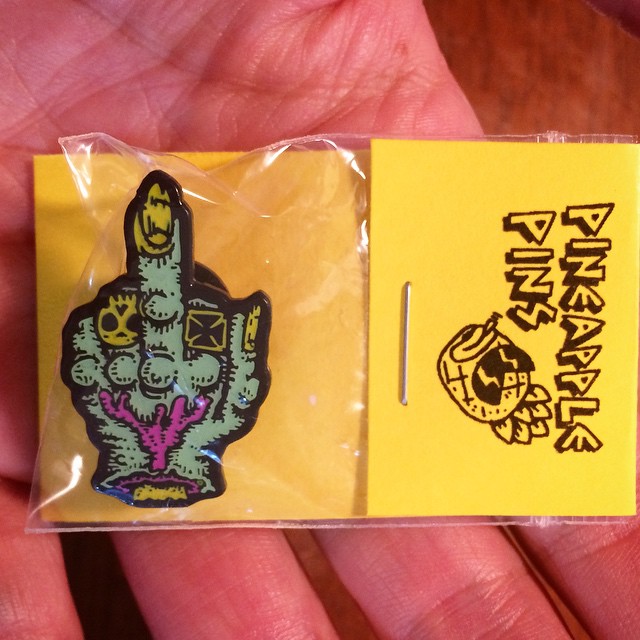This close-up photograph showcases a small, decorative pin designed to be fastened to clothing or accessories. The pin, still encased in its original plastic packaging, is displayed in the palm of a left hand with fingers extended, presenting the package laid on its side. The pin, which appears slightly gory and reminiscent of a zombie hand, depicts a green, lumpy fist with a yellow-painted middle fingernail raised in a vulgar gesture. Notable details include a yellow skull ring on the ring finger and a pink base that resembles sea coral or exposed veins. The packaging features a yellow label with the text "Pineapple Pins" and an amusing logo of a pineapple sporting sunglasses. This visual combination makes for a peculiar yet striking image, emphasizing both the pin's unique design and the playful branding of Pineapple Pins.